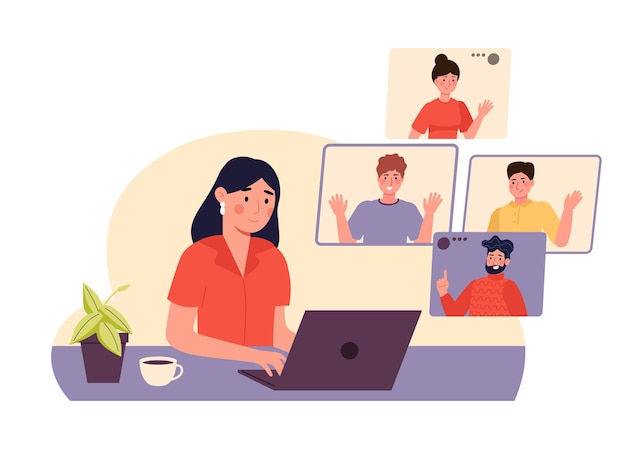In this rectangular, color illustration with a somewhat cartoon-like style, a gray desk spans horizontally across the scene. Seated at the desk is a woman with shoulder-length black hair, wearing a short-sleeved orange shirt. In front of her is an open gray laptop. To her left sits a white coffee cup and a small plant in a black planter. In the upper right-hand corner of the image, there are four small squares, each showcasing a person in a different pose. The lower right square features a man with a beard and black hair, pointing upward with his right hand. Directly above him, in the upper left square, is a young man wearing a gray t-shirt, with both hands held up. Adjacent, in the upper right square, is another young man in a yellow shirt, holding his left hand up as if to wave. At the top square is a female with dark hair in a bun, dressed in an orange t-shirt, similarly raising her left hand in a waving gesture.